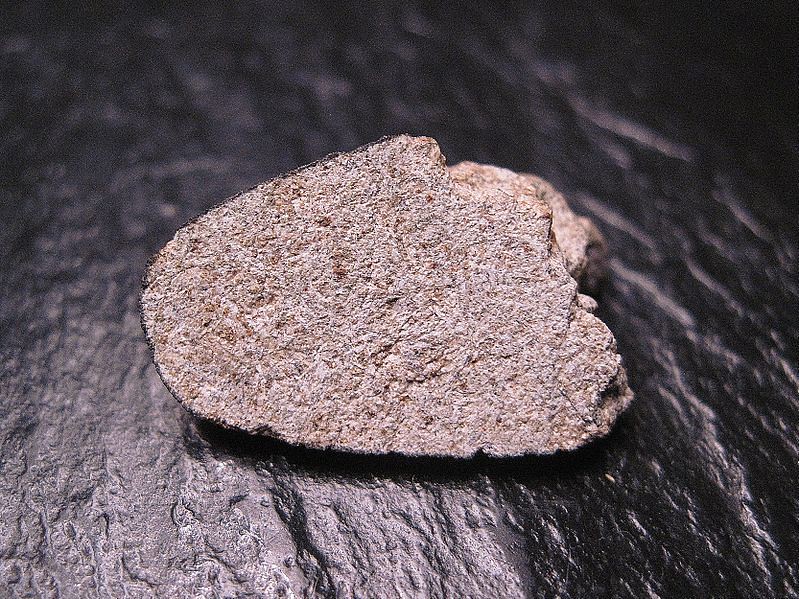This photograph features a smaller, light gray, speckled rock seated atop a larger, smooth, black rock. The focal point is the smaller rock, which has circular form with jagged edges on the upper right side and a smoother circumference on the left and lower side. It is well-lit, displaying speckles of red and teal blue or green. The larger rock beneath it appears very black with smooth, elevated ridges, and it has a shiny texture that suggests a smooth, non-sharp surface. Heavy white lighting from the left side casts a shadow from the smaller rock forward into the foreground, creating a gradient effect on the larger rock, transitioning from light gray on the left to dark gray, almost black, on the right. The background and sides of the image are slightly blurred, sharpening the focus on the central rocks.